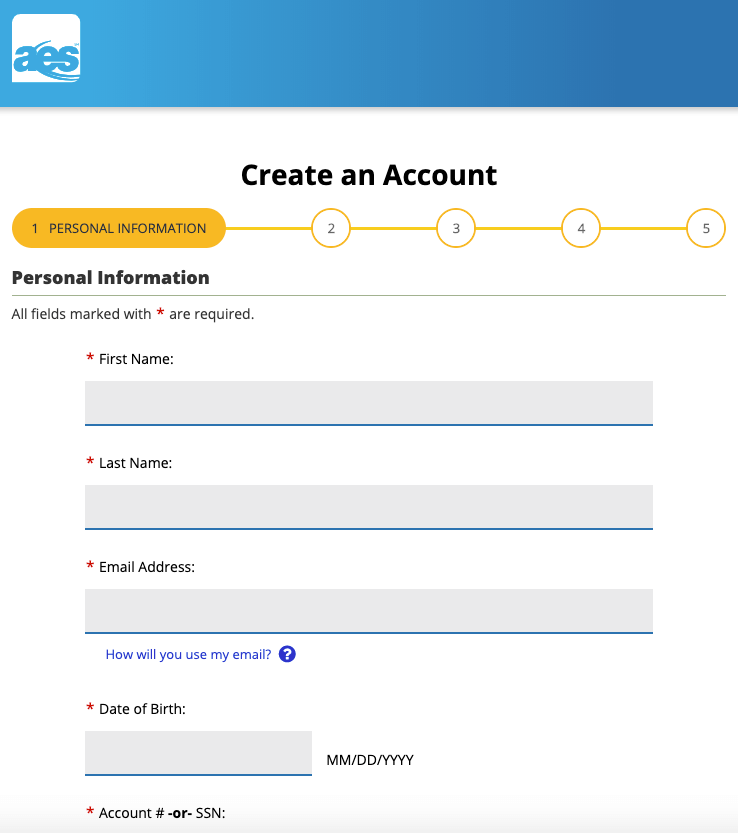The image depicts a user interface for creating an account on a website. At the top of the interface, there is a blue rectangle featuring the AES logo in a white square positioned on the left side. Below this blue header, the background transitions to white, and centered towards the top is the text "Create an Account" in black.

On the left side, there is a yellow rectangle with curved edges labeled "1. Personal Information." This section is connected to subsequent steps via a yellow line that progresses down the interface. Below this first step, there are additional steps marked with numbers inside white circles, bordered by yellow lines: "2," "3," "4," and "5."

Following this sequence, the section title "Personal Information" appears in black text, underlined by a grey line. Beneath this line, the text indicates that "All fields marked with a star are required."

The form is divided into four fields for user input:
1. First Name (marked with a star indicating it is required), with a corresponding input box.
2. Last Name (also required), with a corresponding input box.
3. Email Address (required), with a corresponding input box.
4. Date of Birth (required), with a corresponding input box.